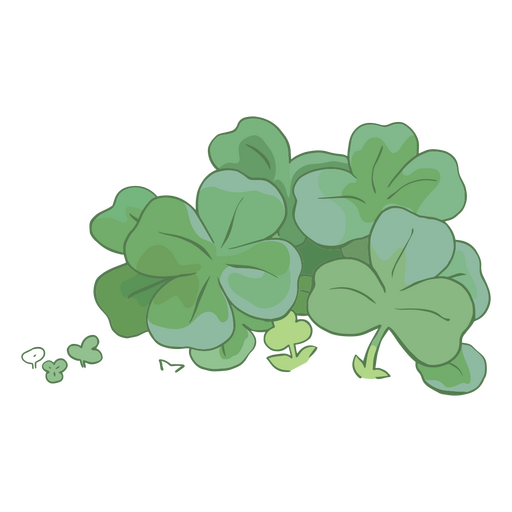This image is a detailed hand-drawn or digital illustration of various three-leaf and four-leaf clovers displayed on a plain white background. There are five to six prominent clovers situated centrally, rendered in a range of green shades from light to dark, giving a watercolor effect. Surrounding the central clovers, mainly towards the edges, are smaller clovers presented in both green and white. Notably, one smaller three-leaf clover in the middle has a distinctive yellow hue. A few clovers show visible stems, which are slightly yellowish. Overall, this artistic depiction of clovers captures a vivid gradient of green tones, creating a visually pleasing contrast with the blank white backdrop.